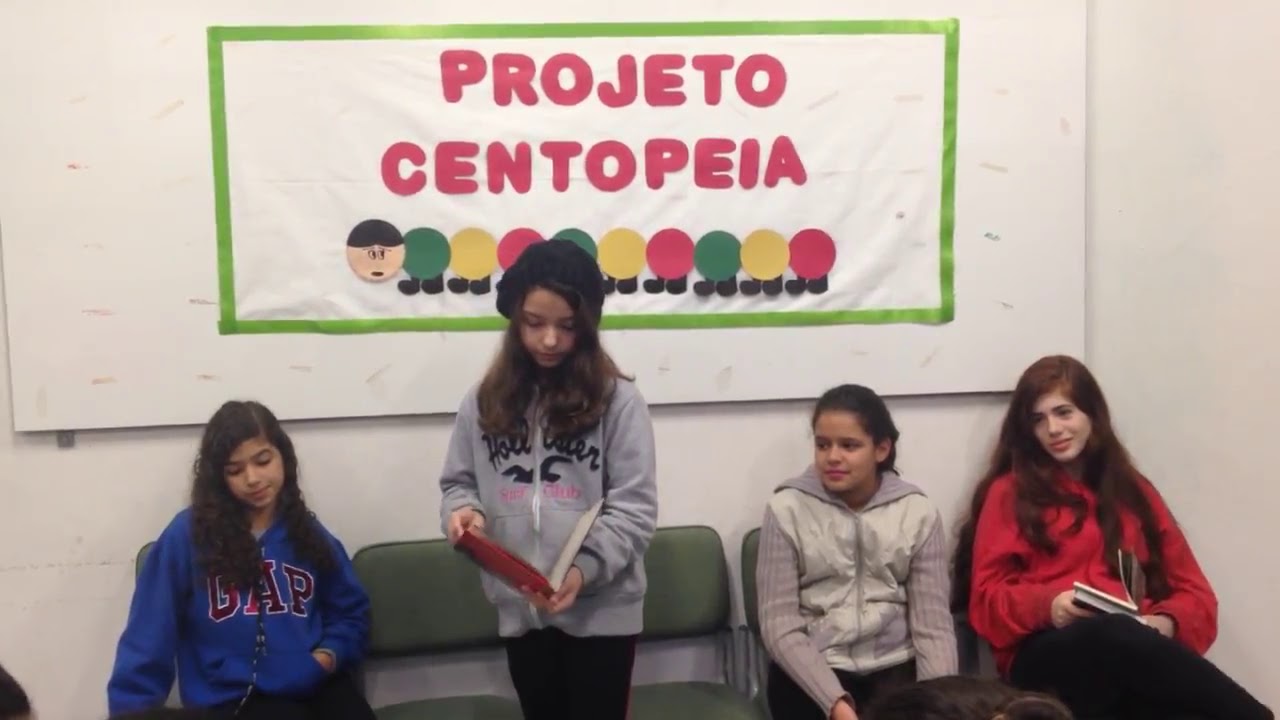This indoor photograph captures a group of four teenage girls, seemingly aged 13 to 14 years, in a waiting room with white walls. The background wall features a banner with a light green rectangular frame and a white center bearing the red-lettered words "Projeto Centopeia." Below the text, there's a row of alternating colorful circles in green, yellow, and red, alongside a cartoonish circular face with dark hair, eyes, and an open mouth.

In the foreground, four green chairs are arranged in front of the banner. Three of the girls are seated while one girl stands, holding and reading from a red-covered book. The leftmost seated girl appears to be around 13, with long dark brown hair, wearing a blue GAP hoodie, and has her left hand in the hoodie pocket while her head tilts slightly to the right as she looks down.

Beside her, the girl standing in the center wears a gray sweatshirt with indistinguishable black writing and black pants. Her long dark hair, partially obscuring the writing on her hoodie, falls well over her shoulders. She also sports a black cap and holds a red-covered book or folder, gazing intently at it.

To her right, another seated girl with brown hair pulled back wears a light gray hoodie with a white puffy vest over it and black pants. She looks towards the standing girl. Finally, the rightmost seated girl in a red hoodie, black pants, and long brown hair also looks towards the standing girl. Her head is tilted to the right, and she holds two books on her lap, with her left leg crossed over her right leg. The girls' focused expressions and casual yet attentive postures indicate a moment of quiet anticipation or concentration in the waiting room.